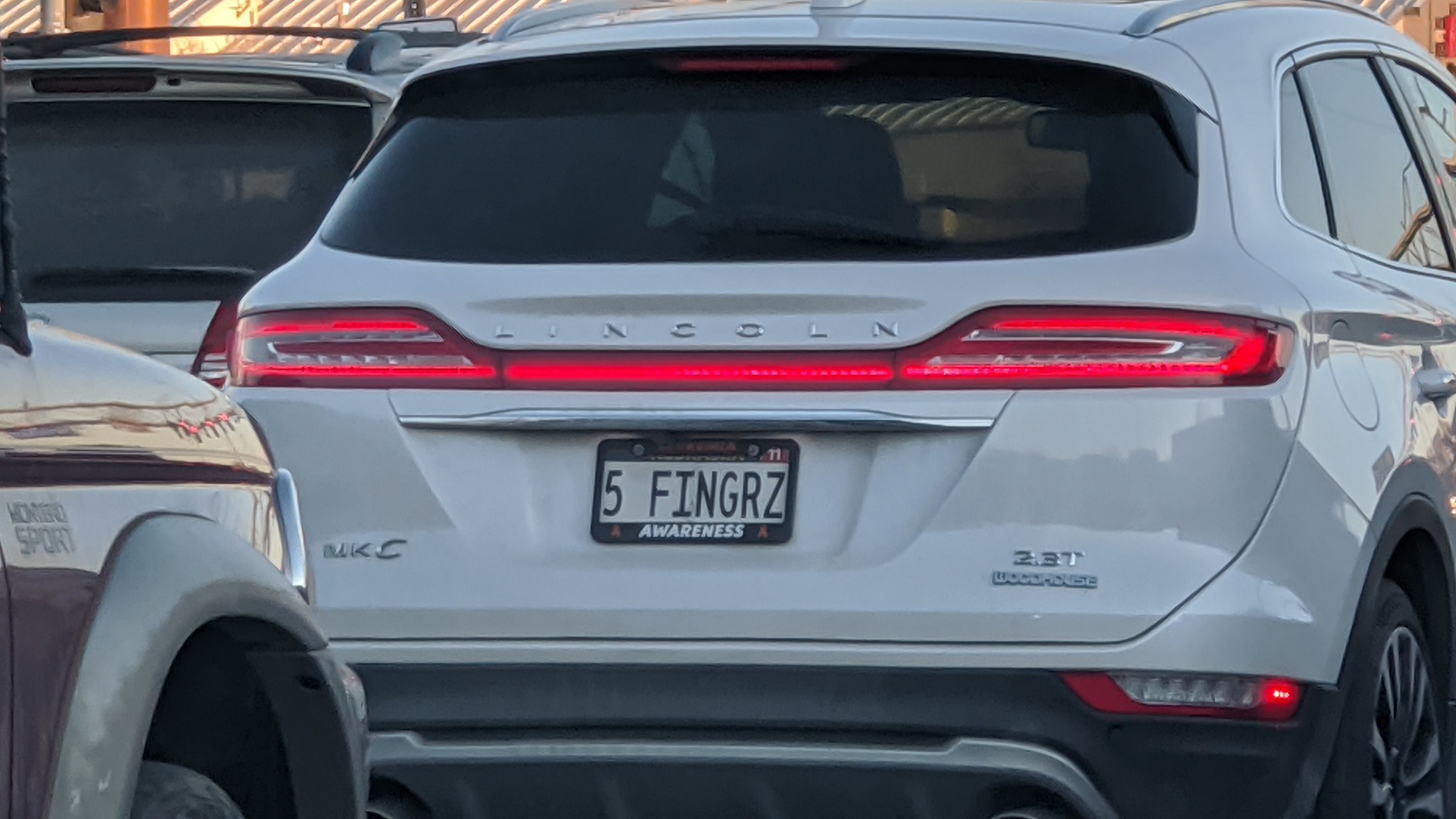This close-up photograph captures the rear of a white Lincoln MKC SUV, prominently displaying the brand name in silver along with the model designation "MKC" on the back left corner and "2.3T" on the bottom right. The license plate, encased in a black frame with the word "Awareness" inscribed in white letters, reads "5FINGRZ" in green text. The vehicle features red brake lights, stainless steel or chrome accents, and a reflection on the right bumper that reveals the surrounding parking lot. In the background, partially visible to the left, is a maroon car with a plastic, light gray wheel well and a black tire, identified as a Mitsubishi Montero Sport by the "Montero Sport" text on its side. The image was captured in mid-afternoon, transitioning toward evening.